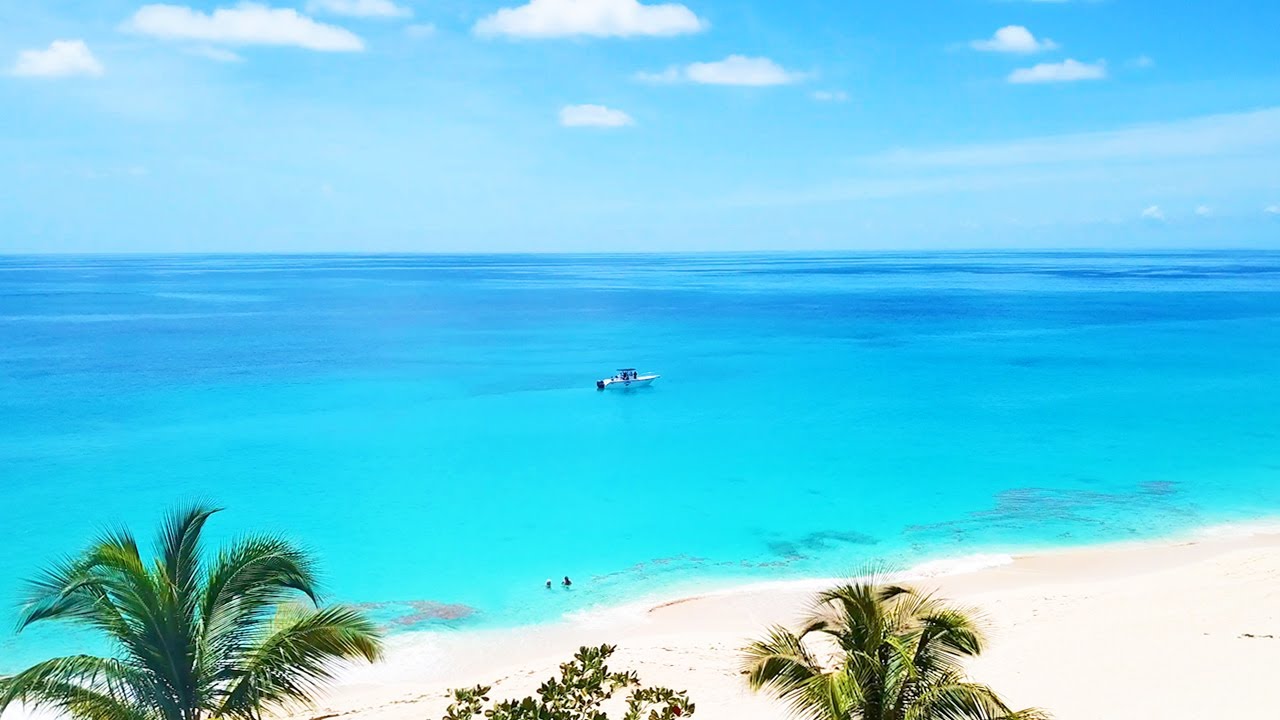This captivating photo captures a serene beach scene under a brilliant blue sky with a few delicate white clouds. The expansive view showcases a turquoise-to-blue gradient ocean, with gentle waves lapping at the pristine white sandy shore that is edged with a foamy surf. At the center of the ocean, a white boat floats peacefully, carrying people who appear tiny from the distance, adding a sense of scale and tranquility. In the foreground on the left side of the image, three tall palm trees stand gracefully with their fronds swaying in the gentle breeze, framing the idyllic setting. Additionally, the upper portions of two more palm trees and a leafy tree with multiple branches are also visible, contributing to the tropical ambiance. The bright and sunny day enhances the vivid colors, making this scene an epitome of paradise.